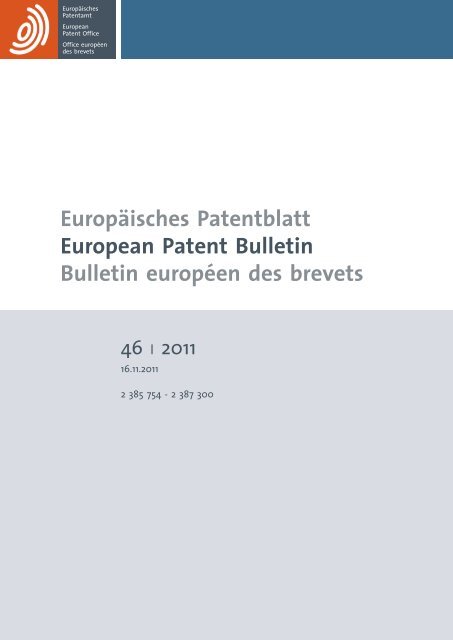The image depicts the front page of the European Patent Office bulletin, presented in three languages: English, German, and French. At the top of the image, against a header backdrop, there is an orange square featuring a logo resembling a stylized white fingerprint with a whorl design. Adjacent to this logo, to the right, is a blue rectangular color block. 

Centered on the page is the title "European Patent Bulletin" written in bold black letters, flanked above and below by the same title in German and French in lighter gray text. Below the titles, in a large light green-gray color block, are various sequences of numbers. The largest numbers display "46" followed by a vertical line and "2011." Below this, in a smaller font, is the date "16.11.2011" (corresponding to November 16, 2011). Further down, in an even smaller font, is another sequence reading "2385754-2387300."

The overall layout is simple, yet organized, with clear demarcations of information through the use of color blocks and different font sizes, ensuring the data is easily legible and distinctly presented.